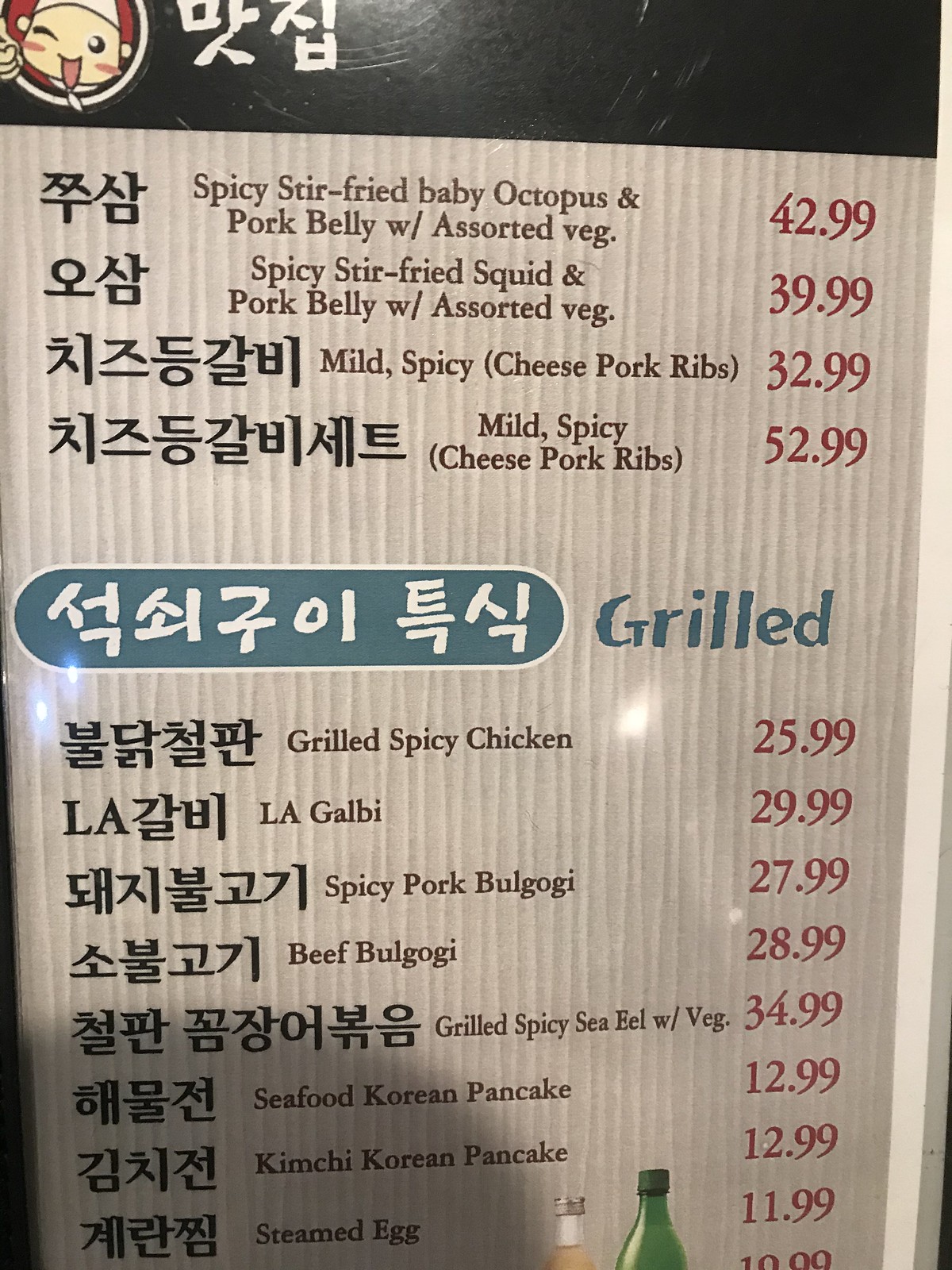The image captures a Korean menu with a distinct design. The top of the menu features a black strip adorned with a small logo and white Korean characters. Listed below, four dishes are prominently displayed: Spicy Stir-fried Baby Octopus, Spicy Stir-fried Squid, Mild Spicy Cheese Pork Ribs (mentioned twice). Following this section, additional Korean text introduces another category titled "Grilled," under which various items are listed: Grilled Spicy Chicken, LA Galbi, Spicy Pork Bulgogi, Beef Bulgogi, Grilled Spicy Sea Eel with Vegetables, Seafood Korean Pancake, Kimchi Korean Pancake, and Steamed Egg. All the dish prices are highlighted in red along the right side. At the menu's bottom, partial images of a soda bottle and what appears to be a wine bottle are visible. The bottom-left corner of the picture is shadowed, likely by someone's head or the camera/phone taking the image.